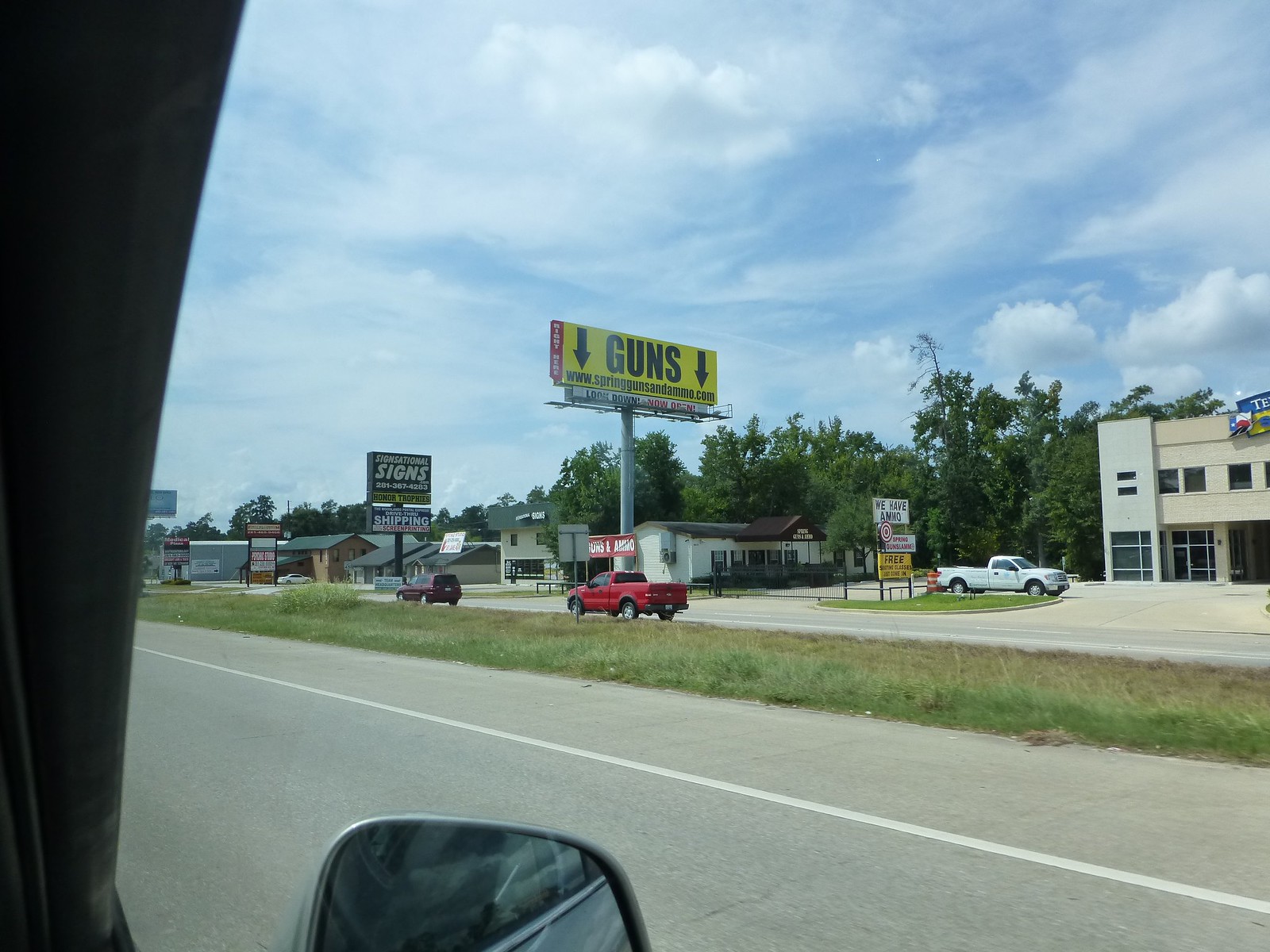This image, taken from the passenger side of a car, captures an outside scene on an average American road. The viewer looks through the car window, with part of the car frame and the right side mirror visible at the bottom of the picture. The sky is a vivid blue, dotted with many white, fluffy clouds.

In the foreground, a highway runs parallel to the road with a grassy median that appears in need of mowing. To the right of the median stands a prominent business sign: a large, vertical yellow billboard with bold black text that reads "GUNS" and features two arrows pointing straight down at a small older-style building resembling a long house but clearly a business due to its awning.

Further ahead, another sign announces "Sign National Signs" and "Shipping," indicating businesses related to signage and shipping services. The buildings lining the road are primarily beige or white with gray or brown roofs and are typical of strip mall or office-type constructions. Behind these buildings, a tree line creates a natural backdrop.

Traffic on the road includes a red pickup truck passing by the gun store and a dark red SUV, sometimes appearing more like a crossover or large station wagon, alongside a white pickup truck parked in front of one of the businesses. The scene is framed by the trees and expansive sky, combining elements of commercial activity with natural surroundings.